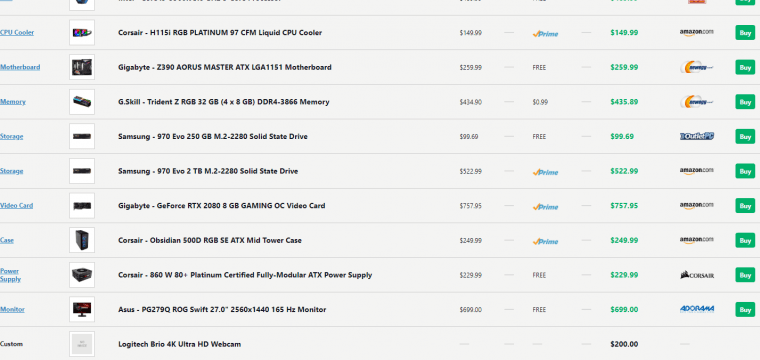A detailed and descriptive caption for this image could be:

"This image features a snapshot from the PCPartPicker website, a popular platform for custom PC builds. While the site name is not visible, it is apparent from the interface that users can select and assemble individual computer components, ensuring compatibility and calculating total costs including shipping. The cropped image shows an array of components selected for a high-performance PC build. Notably, the liquid CPU cooler is a premium Corsair model priced at $140. The motherboard is a Gigabyte Z390, designed for advanced computing needs. The system boasts 32GB of G.Skill Trident memory, providing ample capacity for multitasking and gaming. Storage solutions include a Samsung 970 Evo SSD and an additional 2TB solid-state drive for extensive storage requirements. The graphics card is a powerful Gigabyte GeForce RTX 2080, ensuring top-tier performance for gaming and graphical applications. Additionally, the build includes peripherals such as a webcam and a monitor, rounding out the comprehensive setup."